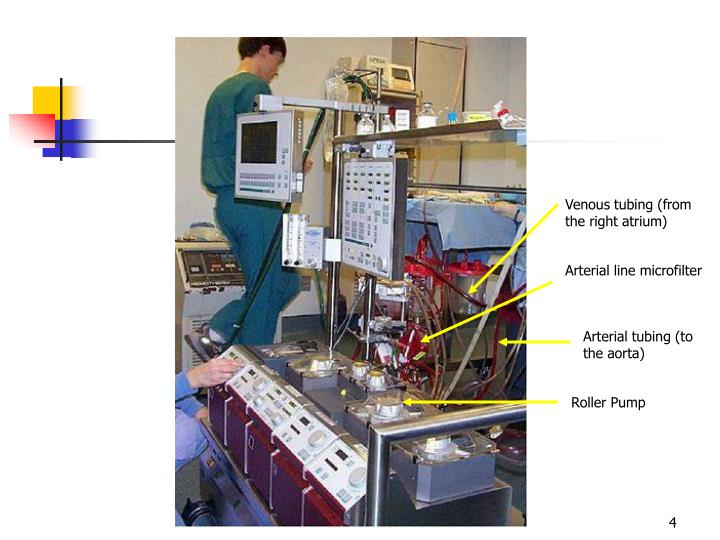The image portrays an older, detailed, and complex piece of hospital equipment set in an emergency room or a similar medical setting. Dominating the image is a sophisticated machine equipped with multiple panels, knobs, dials, and metal support poles. Various components such as venous tubing from the right atrium, an arterial line microfilter, arterial tubing to the aorta, and a roller pump are highlighted with yellow arrows and labeled in black text. A red section at the front of the machine houses many of these controls. To the left, a person's hand is visible, adjusting one of the dials, while another individual in teal scrubs can be seen walking past. Behind this person, another machine and a stark white wall are also visible. The overall atmosphere suggests a preparation or setup phase, perhaps for an upcoming procedure, rendered in what appears to be a slightly dated photograph given the older appearance of the equipment.